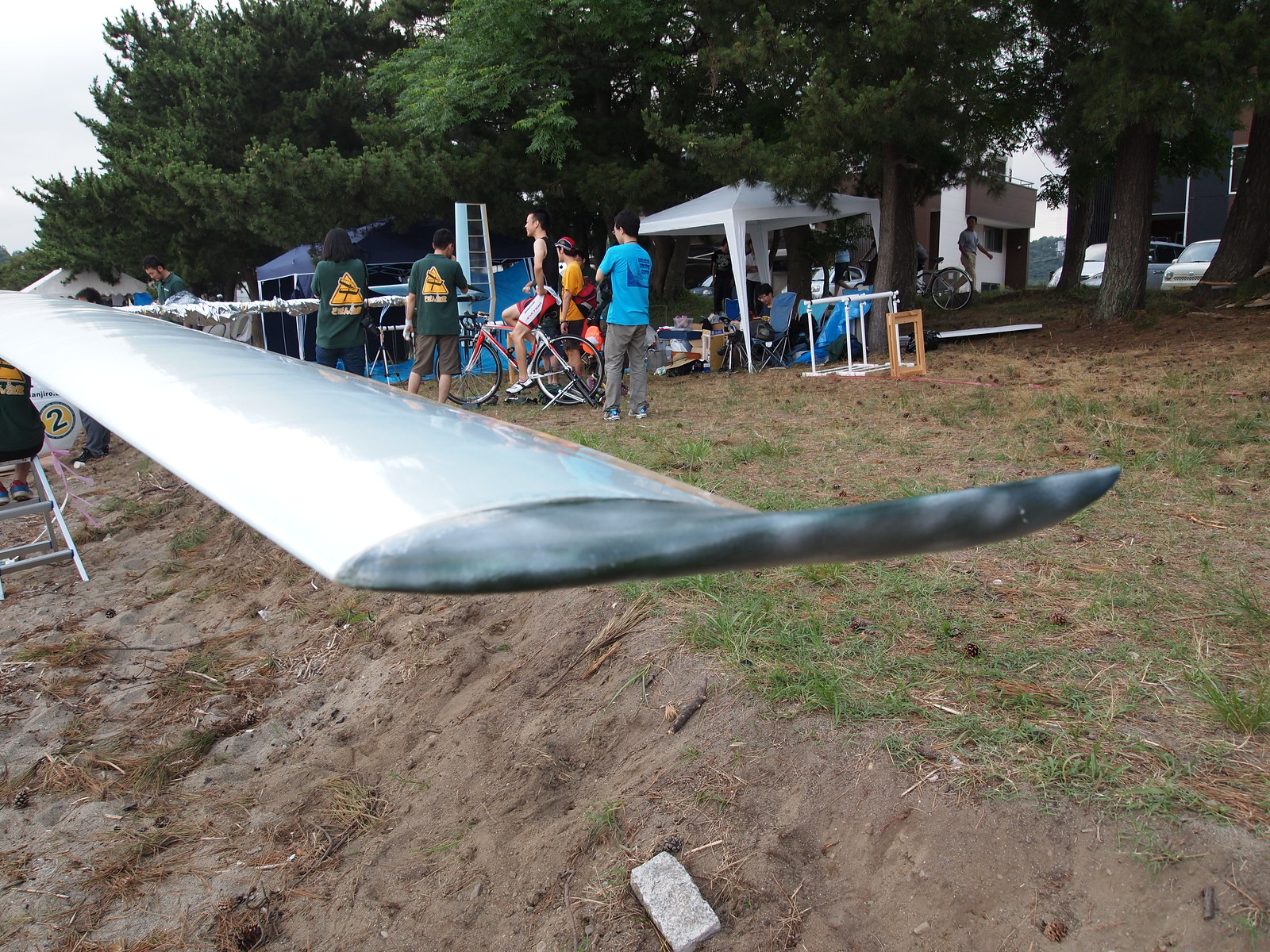The photograph features a bustling outdoor event set on a sloped grassy hill adorned with tall green trees. Prominently in the foreground is a long, slender white object resembling an airplane blade or wing, giving a striking 3D effect. A diverse group of people in colorful attire—green, blue, and yellow shirts—are gathered, some of whom are engaged in discussions, while others are working on the object or nearby. Bikes are scattered around the scene, one notably ridden by a person in a black tank top and red shorts. Tents in blue and white hues are set up beneath the trees, with some individuals attending to various projects within. Additionally, the background reveals a mix of housing units—one blue with brown accents, another brown with white trim—and two parked white cars, a minivan and a smaller car. The sky peeking through the top left is a hazy white. Lastly, amidst the congregation is a figure seated on a silver step stool, presumably supervising the event, adding to the dynamic and vibrant atmosphere.